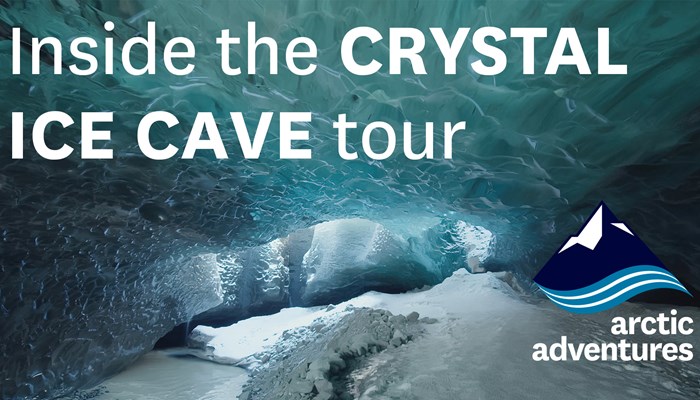This is an advertisement for Arctic Adventures, promoting an "Inside the Crystal Ice Cave Tour." The top of the ad features plain white text reading "Inside the Crystal Ice Cave Tour," with "Crystal Ice Cave" capitalized and bolded. Below this text is an image of a mesmerizing ice cave. The cave has a snowy, frozen floor and a roof of stunning bluish-green ice, showcasing various shapes and textures, almost resembling ripples or waves. The overall scene looks like a serene, frozen underwater world. In the lower right corner, there is the Arctic Adventures logo—a stylized depiction of a mountain or iceberg with a swooping design beneath it, in blue and white. The name "Arctic Adventures" is displayed in bold white text. The image suggests a low-ceilinged passage, adding a sense of adventure and exploration to the tour.